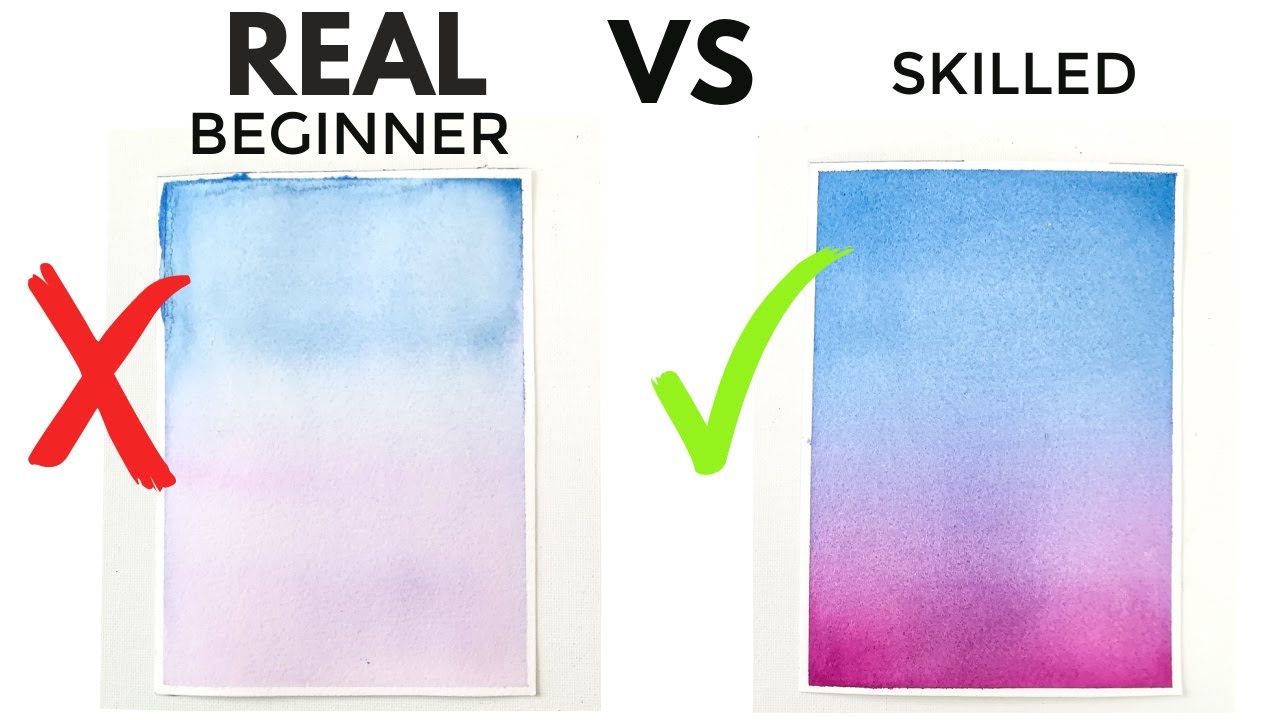This image, set against a white background, features two vertical rectangles side-by-side, each showcasing a blend from blue at the top to purple at the bottom, resembling watercolor on paper. The left rectangle, marked "Real" and "Beginner," is light blue and light purple, with a blotchy and poorly blended appearance. It has a large red X over it. Between the rectangles, the word "VS" is displayed, indicating a comparison. The right rectangle, labeled "Skilled," has a more vibrant and deeper shade of blue at the top and a richer purple at the bottom. This rectangle is well-blended, smooth, and has a large green checkmark. The image contrasts the patchy, lighter beginner's work on the left with the smooth, vibrant skilled work on the right.